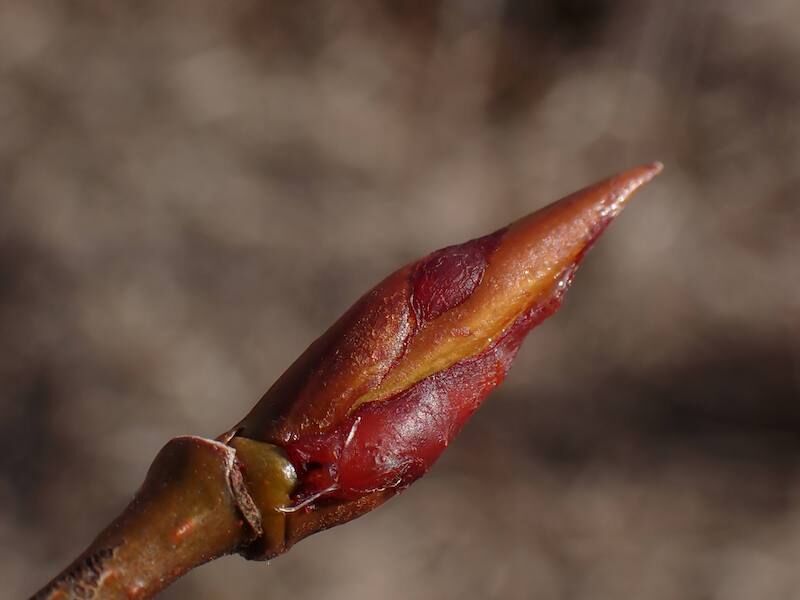This digital photograph captures an extreme close-up of a plant bud poised on the verge of blooming. The focus is on the vibrant tip of the bud, which exhibits a striking mix of red and yellow hues. The bud itself is situated at the end of a thick, dark green stem that emerges from the bottom left corner of the image. Surrounding the plant is a blurred background rendered in soft shades of gray, brown, and subtle hints of white, ensuring that the plant remains the central focus. The background's blurriness not only highlights the intricate details of the bud but also provides a sense of depth and contrasts beautifully with the vivid colors of the plant.